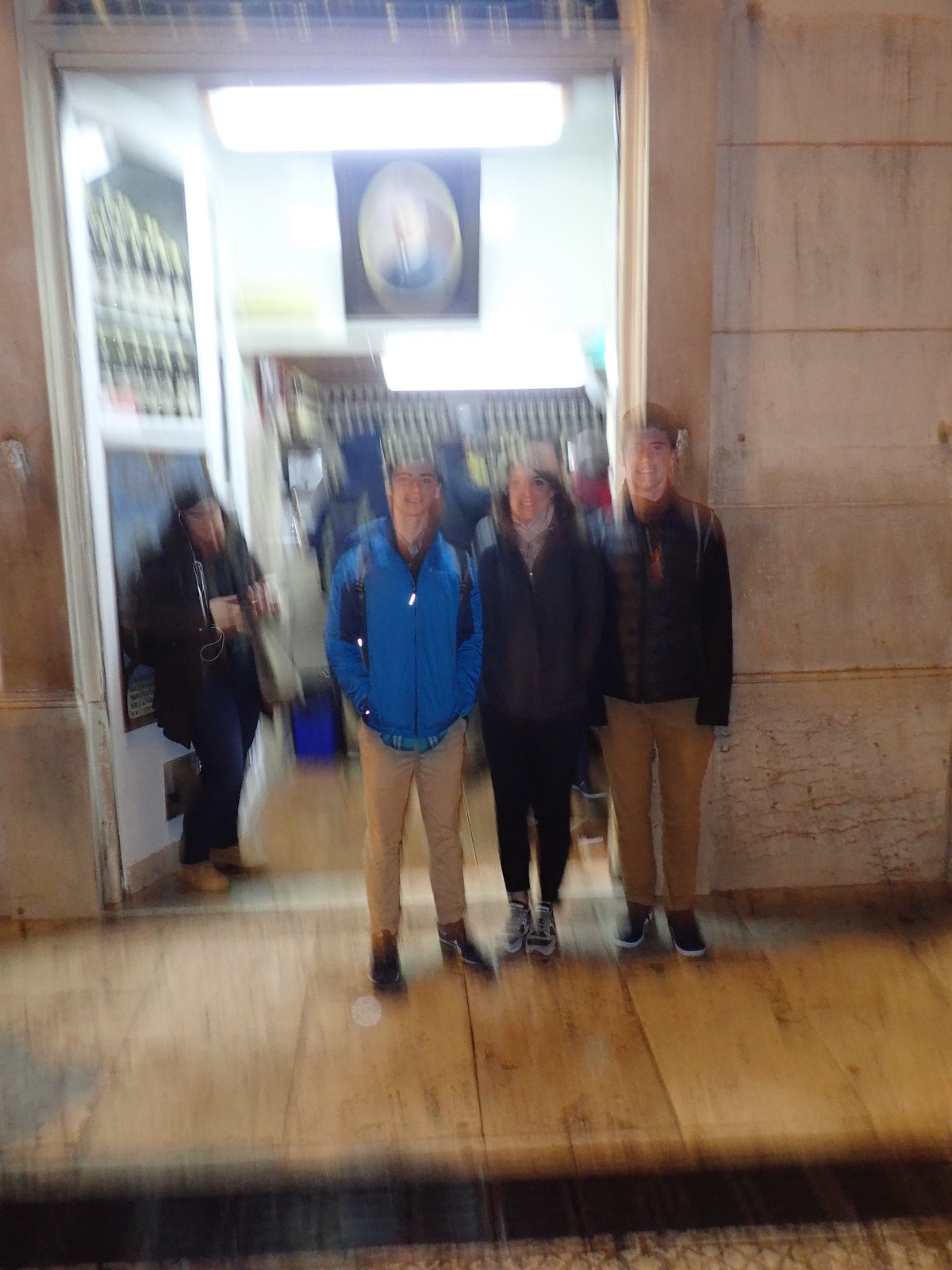The image is a very blurry nighttime color photograph capturing four individuals in front of a brightly lit storefront. The background shows the store's entrance with racks of products faintly visible due to fluorescent lighting. A tiled walkway, indicating an indoor mall setting, leads up to the entrance. In the center of the image on the dark tan sidewalk stand three young people in their early 20s. On the left is a male with his hands in his pockets, wearing a blue jacket and tan pants. The woman in the middle sports a dark jacket, dark pants, and long brunette hair. On the right is a slightly taller man wearing a black jacket, tan pants, and blue sneakers. To the far left, leaning against the entrance door, stands another young woman. The image's high motion blur obscures many facial and finer details, but the scene is well-defined by the contrasting lighting and clothing colors of the subjects.